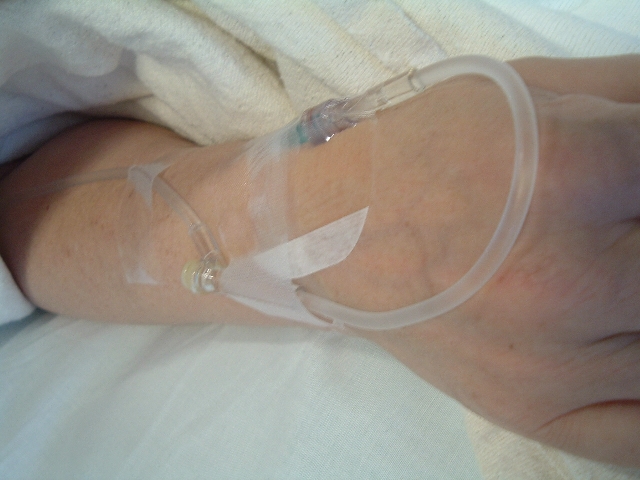The photograph captures a close-up view of a patient's wrist in a medical setting, specifically showcasing the intricate details of an IV insertion. The patient's wrist, exhibiting pale skin with visible blue veins, rests on a white sheet, likely part of the standard bedding in a hospital environment. Their arm appears to emerge from beneath a thicker, wool-like blanket, suggesting they are lying in bed.

A green-tipped needle is carefully inserted into a vein on the right side of their wrist, secured with medical tape. The flexible connection tubing curves around the back of the hand, is meticulously taped at multiple points from the wrist up the forearm, and extends out of the frame, presumably connected to medical apparatus out of sight. The absence of arm hair might hint at the patient being female, although the general texture and paleness of the skin suggest that it could belong to an older individual. The overall composition of the photo underscores the stark and clinical reality of receiving medical care.